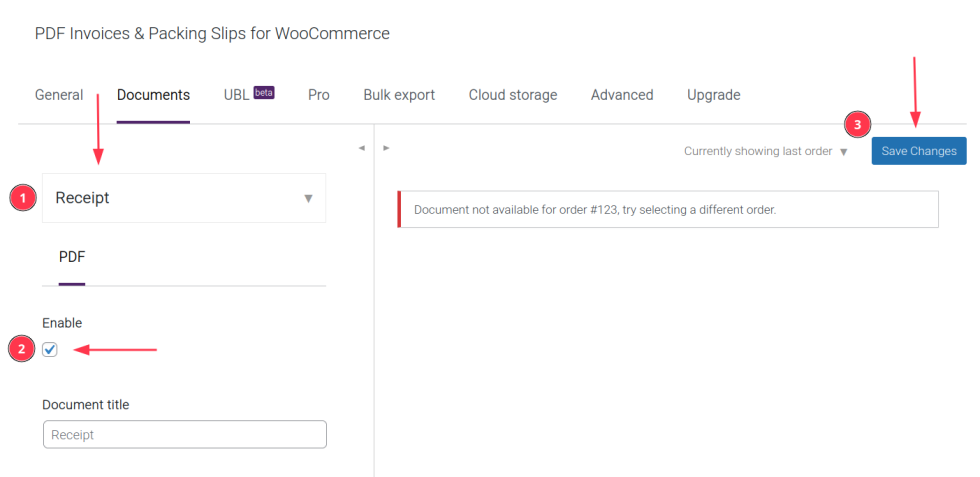Screenshot of a desktop application or website designed for managing WooCommerce invoices and packing slips. The interface features a predominantly white background with sections of black text and various accents. In the upper left corner, the title "PD Invoices and Packaging Slips for WooCommerce" is prominently displayed. Below the title are several navigational options: General, Documents, UBL (marked with a purple beta logo), Pro, Bulk Export, Cloud Storage, Advanced, and Upgrade. The "Documents" tab is currently selected, indicated by a purple underline.

Within the Documents section, there is a drop-down menu labeled "Receipt," which is set to "PDF." To the right of this, there's a checkbox labeled "Enable," associated with the Document Type "Receipt."

A set of instructions is presented, highlighted with red circles and arrows for clarity:
- **Step 1:** Focus on the "Receipt" drop-down menu.
- **Step 2:** Click the "Enable" checkbox.
- **Step 3:** Click the "Save Changes" button, which stands out with white text on a blue rectangle background.

The interface shows an alert for the "Last Order," stating: "Document not available for order number 123. Try selecting a different order." This indicates that the software or application is intended to facilitate business operations, specifically focusing on managing and generating necessary documentation for WooCommerce transactions.